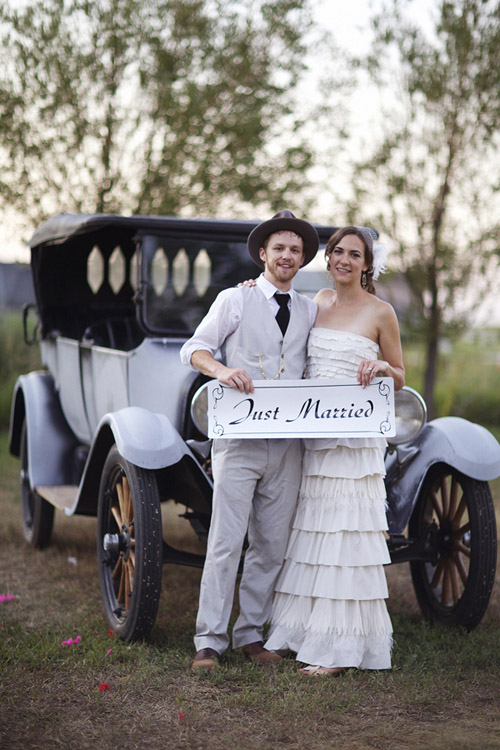In this vibrant daytime outdoor photograph, a joyful newlywed couple stands beaming at the camera, holding a white sign with black lettering that says "Just Married." On the left, the groom, a white man with a stubbly red beard, exudes a vintage charm in his light gray vest and matching slacks, accompanied by a black tie and a white button-down shirt with rolled-up sleeves. His ensemble is topped off with a black hat and casual shoes. To his right, the bride, a white woman with brown hair, looks radiant in a layered, strapless white wedding dress. A delicate, frilly veil or ribbon adorns the back of her hair, adding to her elegant appearance. They are standing in front of a classic gray and black Model T car, its hood just behind them, further enhancing the timeless feel of the scene. Their surroundings include a lush grassy field with scattered red and pink flower petals, tall trees, and a hint of a hazy sky above, indicating an open countryside setting. Their smiles, sincere and filled with happiness, capture the celebratory essence of their special day.